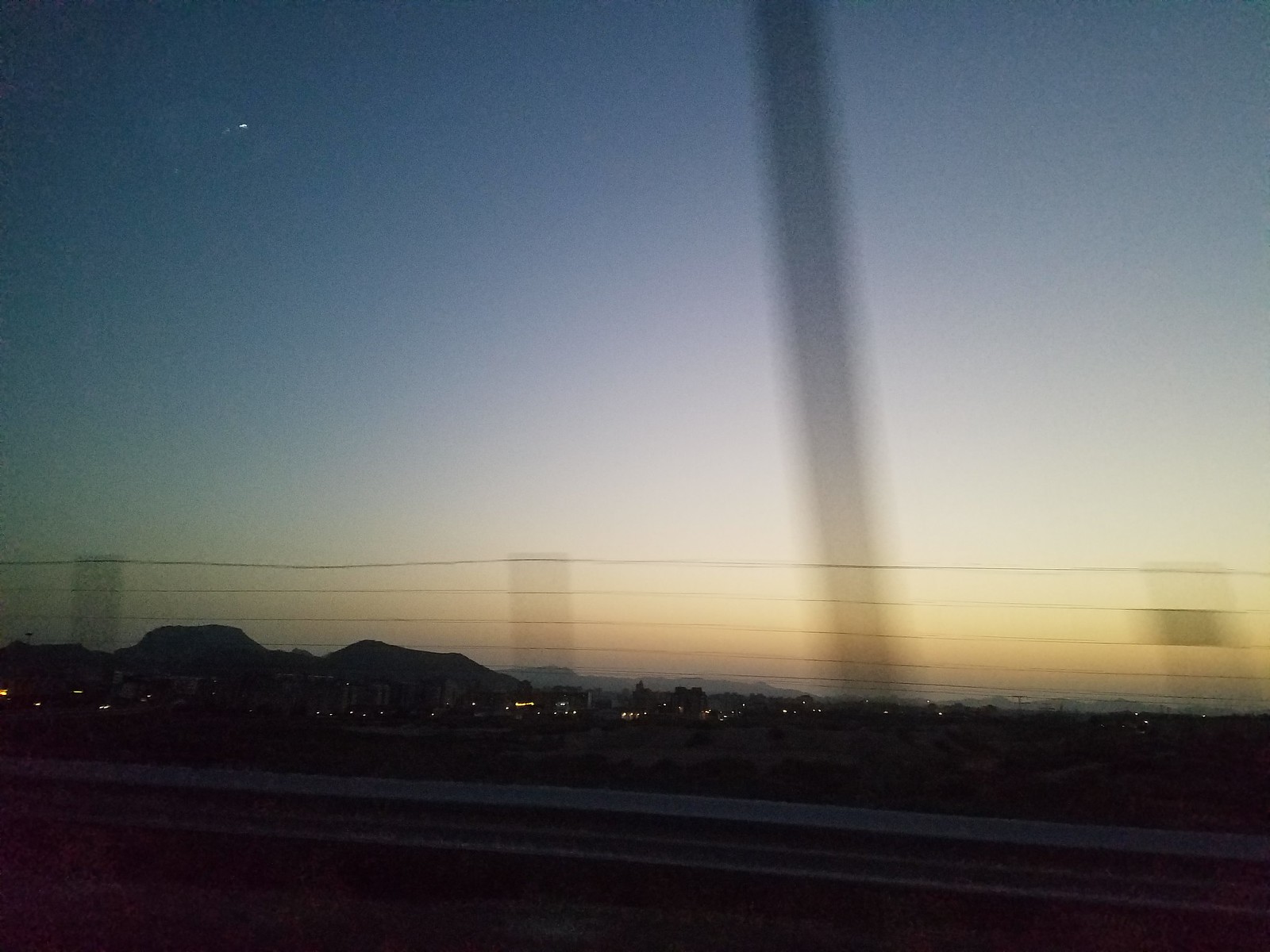This somewhat blurry photograph, possibly taken through the window of a car or a train, captures a hazy dusk or night scene. In the background, the dark night sky gradually transitions into a band of yellowish-orange near the horizon. A shadowy figure of what appears to be a tall pole or lamp post slices vertically down the middle of the image, extending towards the bottom. 

Across the midsection of the photograph, faint horizontal lines resembling a fence stretch from left to right. This fence-like structure might be a reflection on the window rather than an actual part of the scene. Below, towards the bottom, a metal highway barrier or railing runs horizontally along the frame, suggesting the picture was taken from a moving vehicle. 

In the distance, the faint white lights of a small town or rural area twinkle, providing a sparse, desolate ambiance to the landscape. Behind these scattered lights, the silhouette of hills can be discerned, adding depth to the scene. The image, devoid of crowded urban features, conveys a serene, almost isolated feel.